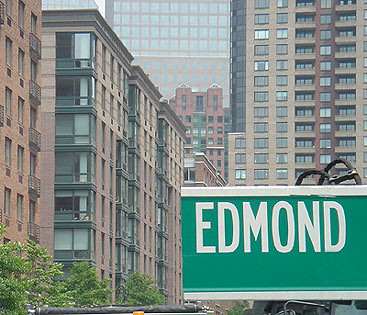The image showcases a cluster of imposing high-rise buildings, each seemingly constructed of concrete and punctuated with numerous windows. These structures are arranged in a rough square formation, creating a sense of architectural enclosure. Prominently featured in the background is one particularly striking building, characterized by an almost unbroken expanse of windows, with four distinct layers stretching across its upper levels. A green street sign with white edges and the name "Edmond" emblazoned in white letters is prominently displayed in the foreground. Adjacent to the sign, black metal elements are visible, possibly part of urban infrastructure. A silver-colored metal fence, likely made from interconnected steel wires, also borders the scene, adding to the urban landscape’s detailed texture.